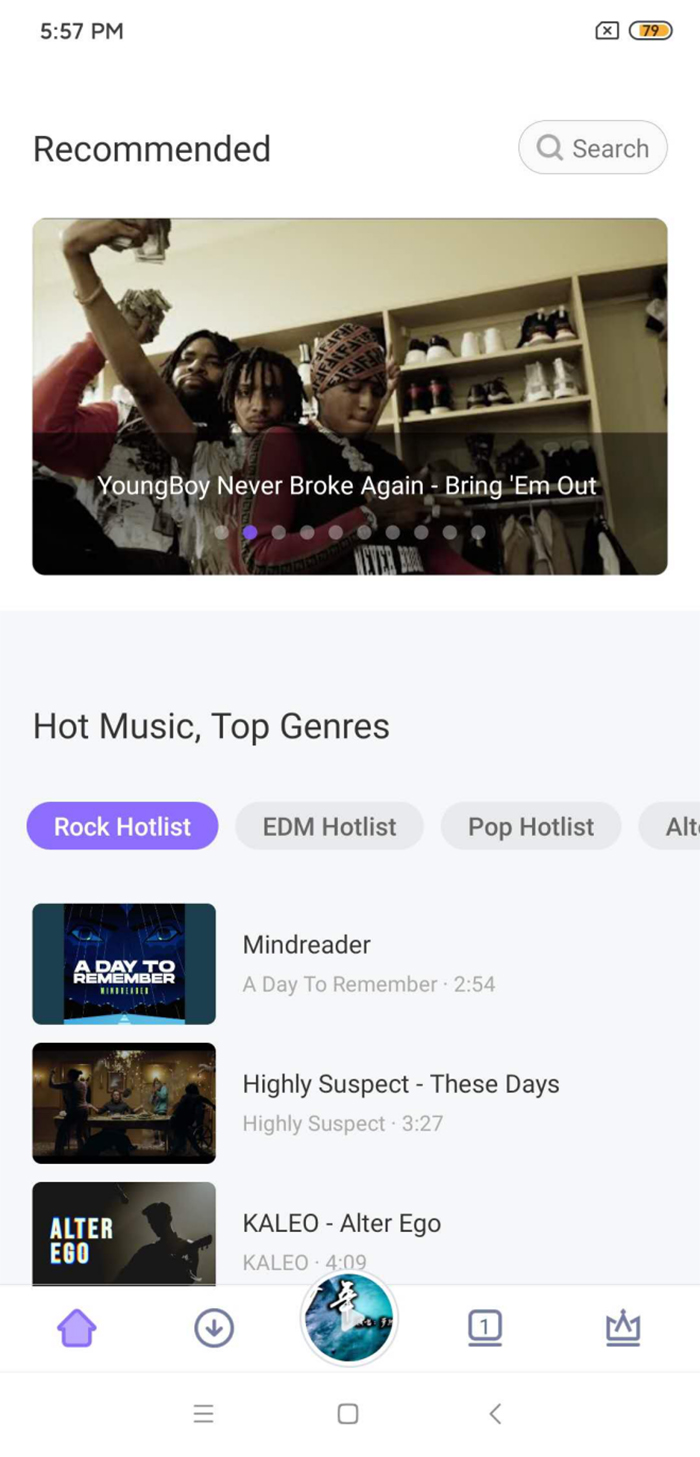The screen capture showcases an application interface with a minimalist, light-colored theme. The background is predominantly white, with certain sections highlighted in lighter gray. The app uses purple as its accent color, while the primary text is a dark gray. 

At the top of the screen, the device status bar shows the current time as 5:57 p.m., with a battery life of 79%. Below this, the app's header reads "Recommended," accompanied by a search bar.

The main header image features a group of young Black men in their early to mid-20s, with a text overlay stating, "YoungBoy Never Broke Again – Bring Him Out." Indications for a slideshow, represented by dots, suggest there are additional header images and recommendations to browse through.

Beneath this, a lighter gray section separates itself from the header. Titled "Hot Music – Top Genres," it offers a range of musical filters, with "Rock Hot List" selected and highlighted in purple. Additional genre filters like "EDM Hot List," "Pop Hot List," and potentially "Alternative" (partially obscured) are shown in lighter gray text.

This section is followed by a list of linked songs and videos, each accompanied by a thumbnail image. The listed songs include:
- "Mind Reader" by A Day to Remember, duration 2 minutes and 54 seconds.
- "These Days" by Highly Suspect, duration 3 minutes and 29 seconds.
- "Alter Ego" by Kaleido, duration 4 minutes and 9 seconds.

Below these entries, the app’s various buttons and navigation options are visible.